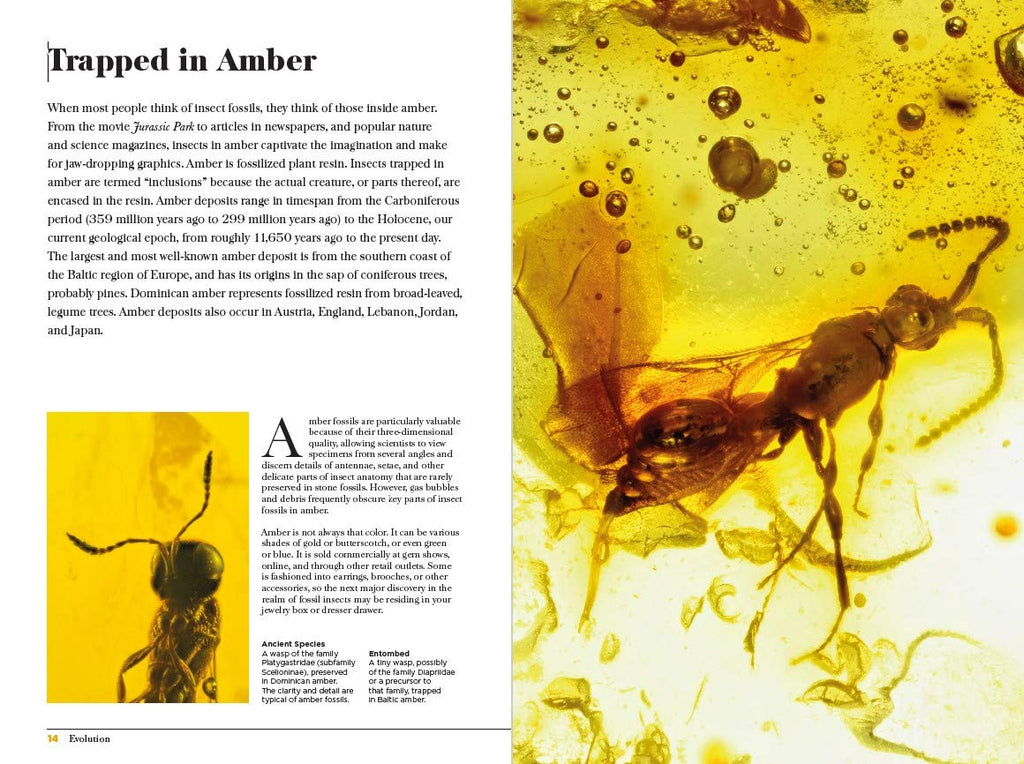This page from a magazine or textbook, labeled "Page 14," features an article titled "Trapped in Amber" on the left side. The text elaborates on the fascinating subject of insect fossils preserved in amber, which is fossilized plant resin. Insects encased in amber, known as inclusions, range from the Carboniferous Period to the present day, capturing the imagination through media like Jurassic Park, newspapers, and science magazines. Notable amber deposits are found along the southern coast of the Baltic region of Europe, originating from coniferous tree sap, likely pines. Other significant deposits include Dominican amber from legume tree resin, and amber from Austria, England, Lebanon, Jordan, and Japan.

On the left side beneath the text, there's a small image of an insect, possibly an ant, trapped vertically in amber against a yellow background. On the right side, there's a larger image of another insect, potentially a mosquito, surrounded by a yellow, bubbly substance with white patches below it.